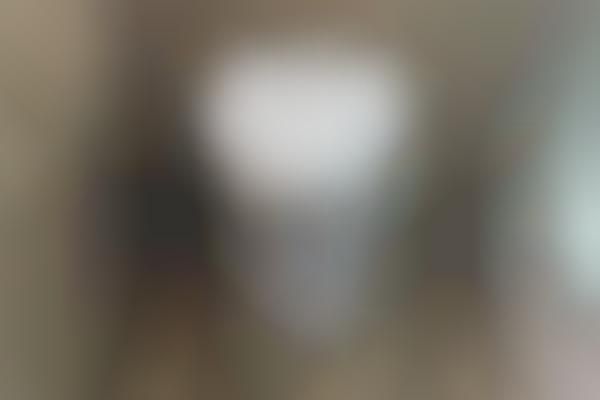This photograph captures a uniquely designed toilet inside an RV bathroom. The toilet features a small, heart-shaped white seat and lacks a traditional tank. Instead, it has a clear tube with white O-rings that connects to the wall on the left side, and a plug that extends through a wall hole. The toilet is equipped with a hand crank on the bottom and a smaller knob on the right side, indicating it may be manually operated or built for specialized use. The lower part appears to be detachable, possibly for waste separation, with a bucket likely intended for dry solids. Adjacent to the toilet is a silver, stainless steel trash can with a foot lever, positioned under the tube. The bathroom floor is covered with wood grain vinyl tiles, and the walls have a grayish textured wallpaper. On the right side of the photo, part of a circular-shaped shower with slightly curved glass sliding doors is visible.